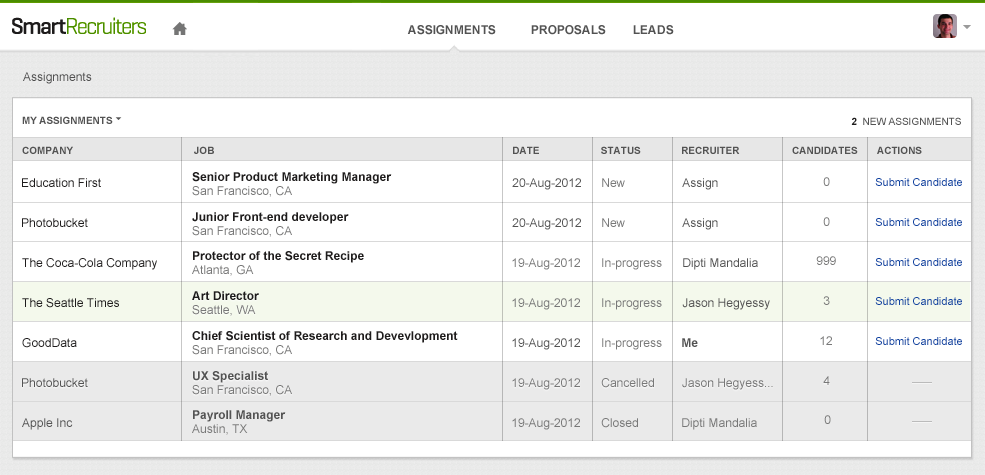**Detailed View of a SmartRecruiters Assignments Page**

The screenshot captures the "SmartRecruiters" platform interface. At the top, there's a prominent white bar featuring three menu options. Within this bar, aligned to the far right, there is a user's profile picture along with a drop-down menu for account settings or additional options.

Below this bar, the active page highlighted is "Assignments," as indicated by the gray navigation bar which clearly states "Assignments" followed by a sub-heading "My Assignments."

The "My Assignments" section is systematically broken down into several columns, providing specific details for each assignment. These columns are labeled as: Company, Job, Date, Status, Recruiter, Candidates, and Actions.

1. **Education First**
   - **Job**: Senior Product Marketing Manager
   - **Location**: San Francisco, California
   - **Date**: August 20th, 2012
   - **Status**: New
   - **Recruiter**: Assigned
   - **Candidates**: 0
   - **Action**: Submit Candidate

2. **Photobucket**
   - **Job**: Junior Front-End Developer
   - **Location**: San Francisco, California
   - **Date**: August 20th, 2012
   - **Status**: New
   - **Recruiter**: Assigned
   - **Candidates**: 0
   - **Action**: Submit Candidate

3. **Coca-Cola Company**
   - **Job**: Protector of the Secret Recipe
   - **Location**: Atlanta, Georgia
   - **Date**: August 2012
   - **Status**: In Progress
   - **Recruiter**: Dipty Mandela
   - **Candidates**: 999
   - **Action**: Submit Candidate

4. **Seattle Times**
   - **Job**: Art Director
   - **Location**: Seattle, Washington
   - **Date**: August 2012
   - **Status**: In Progress
   - **Recruiter**: Me
   - **Candidates**: 12
   - **Action**: Submit Candidate

Aside from the active assignments, there are also two assignments marked as canceled. These canceled entries are highlighted in gray, indicating their current non-active status.

This detailed breakdown provides a comprehensive overview of the Assignments interface on the SmartRecruiters platform, highlighting the key elements and statuses of various job assignments.